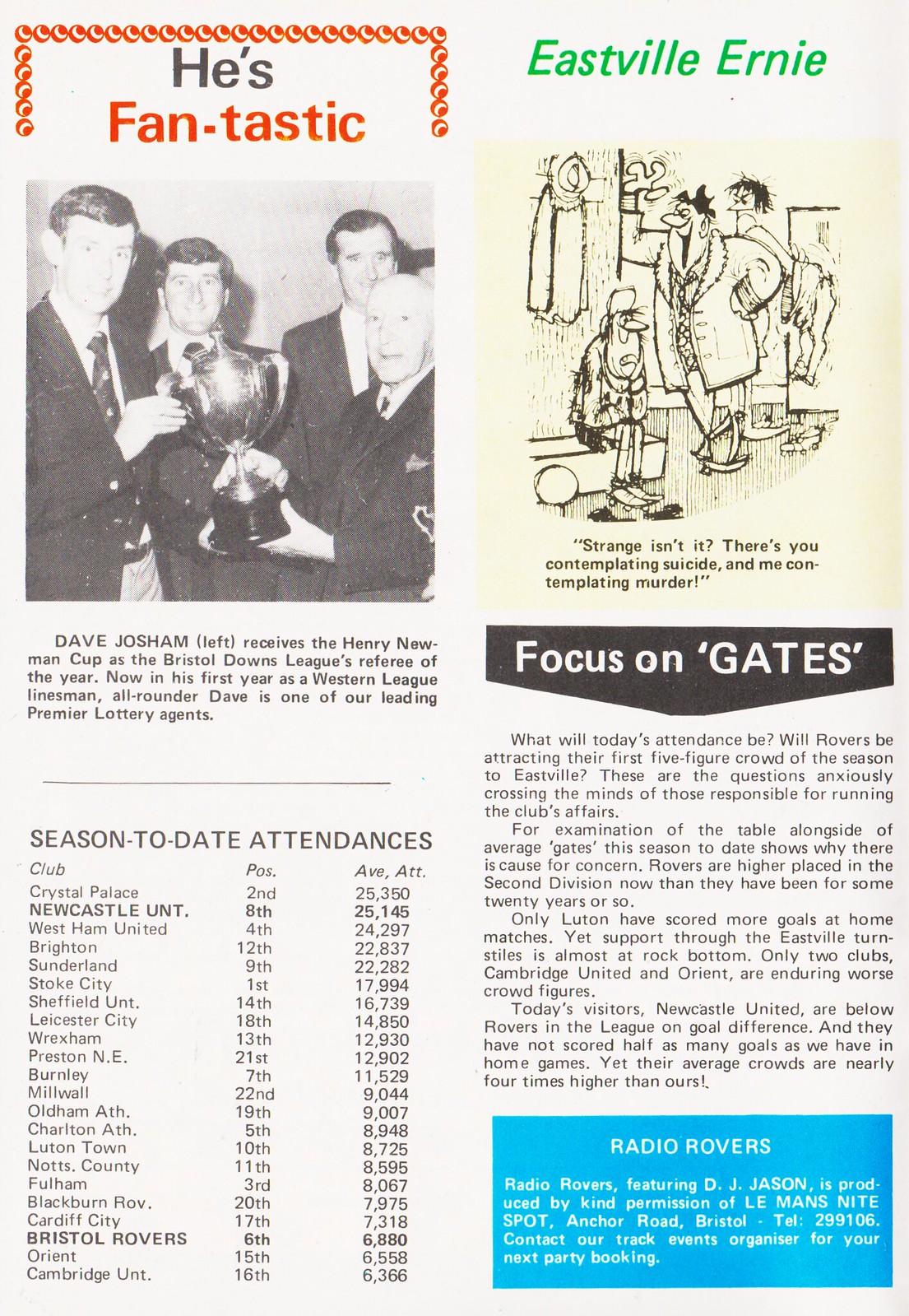The image, likely part of a brochure or magazine, is arranged on an off-white background with two columns. In the top left corner, there is a black-and-white photograph of four men receiving a trophy. Above this picture, the caption reads "He's Fantastic" with "fantastic" highlighted in orange-red font. This picture caption is followed by detailed text stating: "Dave Thompson (left) receives the Henry Newman Cup as the Bristol Downs League referee of the year. Now in his first year as a Western League linesman, all-rounder Dave is one of our leading Premier Lottery agents." Beneath this text, there is a data list summarizing "Season to date attendances listed by club position and average attendance."

The right column features the heading "Eastville Ernie" in green letters above a small black-and-white comic strip. The comic strip humorously depicts a character contemplating serious actions with the text: "Strange, isn’t it? There’s you contemplating suicide and me contemplating murder." Below the comic strip is a detailed paragraph in black font. At the very bottom right corner, there is a rectangular blue box with white text inside, reading "Focus on Gates" followed by a related paragraph.